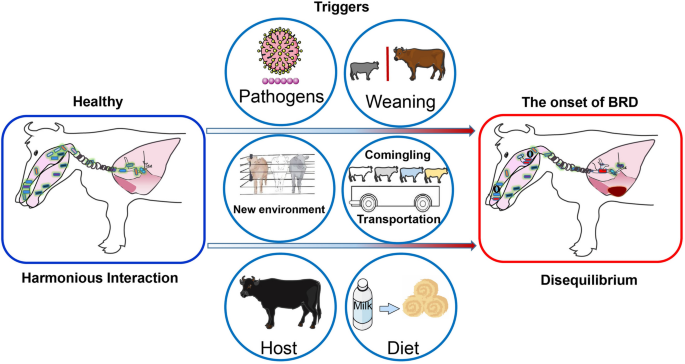This is a detailed diagram illustrating the onset of Bovine Respiratory Disease (BRD) in cattle, presented on a plain white background. On the left, there is a blue-bordered, side-view illustration of a cow showing its mouth and stomach. The stomach appears pink with green enzymes, labeling it as "healthy" with "harmonious interaction" written beneath. Two arrows labeled "triggers" lead from this blue box to a red-bordered box on the right. This section also features a side-view of a cow's stomach but with dark red areas, indicating "the onset of BRD" and "disequilibrium."

Central to the diagram are three descending columns of circles, each with blue outlines and various labels. The top two circles are labeled "pathogens" and "weaning," showing a cow and a calf. The middle circles read "new environment" and "commingling transportation," illustrated with corral fencing and a group of cows with a truck. The bottom circles are labeled "host" and "diet," depicted with a black bull and a combination of milk and hay bales. These elements collectively represent the potential triggers leading to the disequilibrium shown on the right.